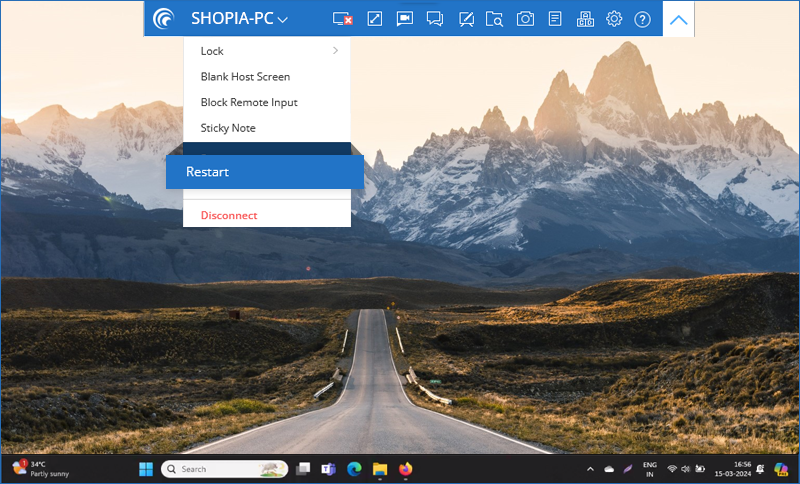The image, sourced from a website page titled "Shapia-PC," prominently displays its name in a top blue rectangle, which also houses clickable icons resembling speech bubbles. These icons include a magnifying glass, a camera, a settings gear, and a question mark. Below this banner, a drop-down menu features various options such as "lock," "blank host screen," "black remove input," "sticky note," "restart," and "disconnect." Notably, the "restart" option is presented in a three-dimensional blue box, matching the primary blue of the top banner, while "disconnect" is highlighted in bold red text.

The central portion of the image showcases a picturesque road leading northward towards distant mountains. These mountains, composed of rugged stone, are capped with patches of white snow. The background is graced by a beautifully illuminated sky, which enhances the scenic nature of the photograph.